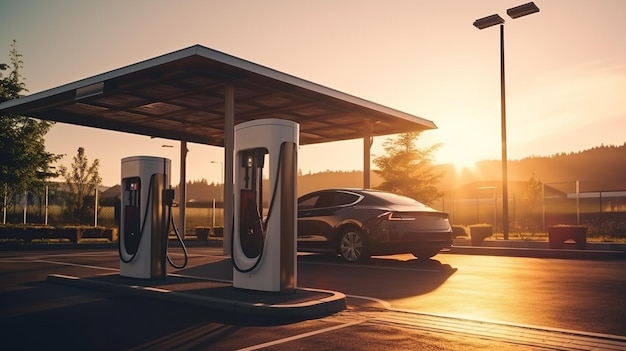The image depicts a futuristic or AI-generated scene at a gas or charging station under a modern carport with two sleek, white pumps equipped with hoses. Central to the image is a dark-colored, modern-looking car, possibly a Tesla, parked to the right of the pumps near a bench on a small grassy patch. The setting appears to be late in the afternoon or at sunset, casting a golden-amber hue over the scene. The sunlight, either rising or setting, illuminates the dry, reflective pavement, emphasizing the clear, vibrant atmosphere. In the background, a tall parking lot light with dual rectangular lamps stands unlit due to the daylight. Surrounding the station are trees, shrubs, and a fence that encloses the area. The overall image conveys a serene and futuristic ambiance with no people visible.